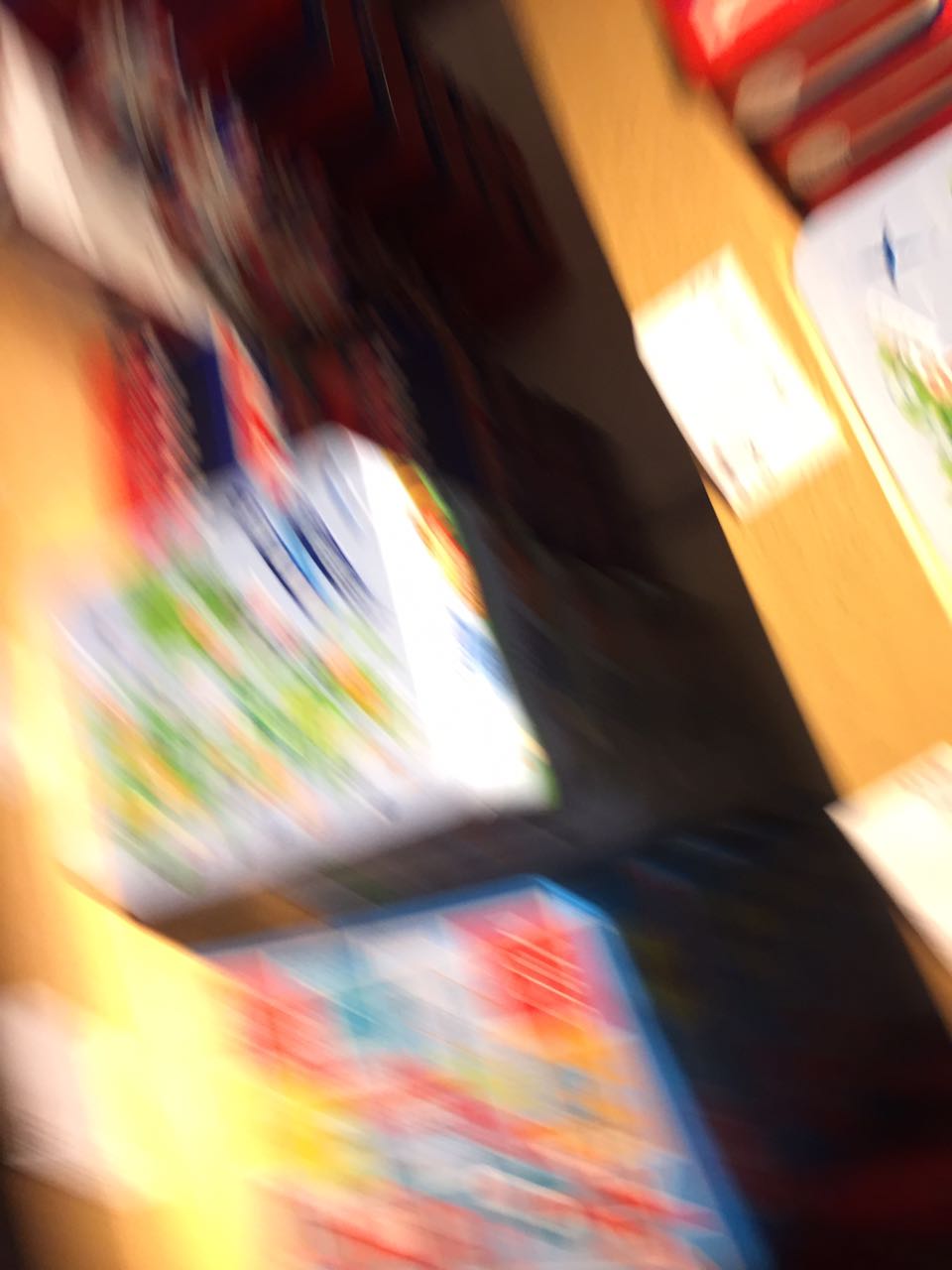The image is notably out of focus, making it difficult to discern precise details. However, it appears to feature an assortment of boxes in varying colors and shapes. Towards the center, there seems to be a rectangular box in a yellow-brown hue. To the left side of the image, another box is visible, though its details remain indistinct. Beneath these, there is a collection of additional boxes that display blue and red colors, accented with occasional yellow. Among the assortment, white boxes are present, one of which may bear a blue logo or design, though the blur obscures specifics. The ground appears to be a white floor, hinted at by patches of white visible near the bottom of the image. Additionally, a stack of red boxes is distinguishable amidst the blurred composition.